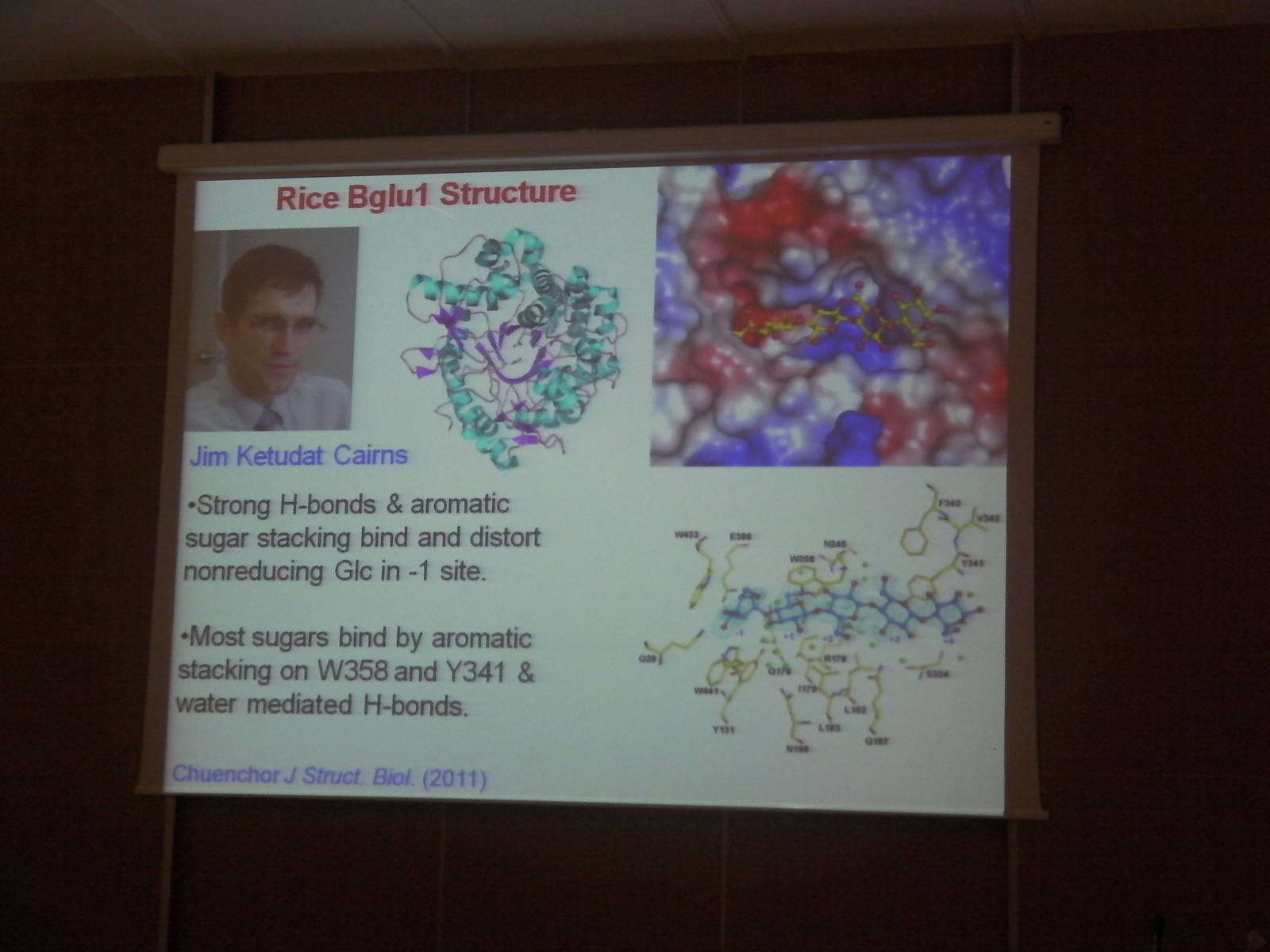This is a detailed photograph of a projector screen, likely in a science professor's classroom, displaying a PowerPoint slide. The slide has a white background with the title "Rice BGLU1 Structure" in red letters at the top. Below the title, on the left side, there's a headshot of a man identified as Jim Ketudat Cairns, written in blue text. The man's headshot shows a white male, with brown hair, glasses, and wearing a white button-down shirt with a tie.

To the right of the photograph, the central part of the slide features several colorful biological diagrams. One diagram depicts intricate molecular structures with colors such as seafoam and purple, blue and red, and yellow and blue, all marked with black labels. Additionally, there is a detailed 3D composite image in the top right corner, displaying red, white, and blue elements, which likely represent molecular bonds.

The left side of the slide also contains two bullet points elaborating on the Rice BGLU1 structure:
1. "Strong H-bonds and aromatic sugar stacking bind and distort non-reducing GLC in negative one site."
2. "Most sugars bind at aromatic stacking on W358 and Y341 and water-mediated H-bonds."

These annotations provide insights into the chemical bonds and interactions within the structure. The overall layout, coupled with the scientific content, suggests that this image is part of a comprehensive biology presentation.